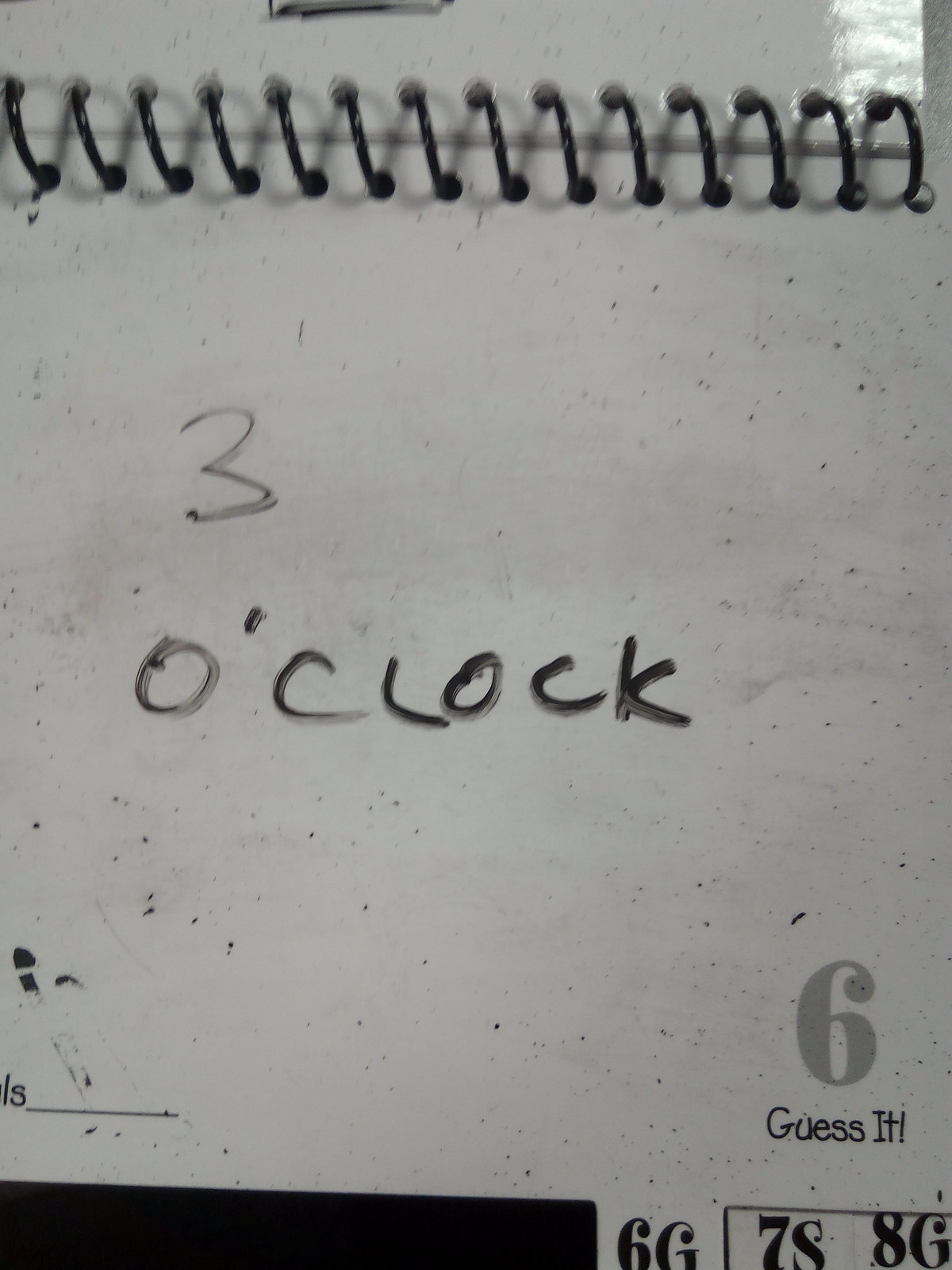The image features a close-up of an unconventional flip pad designed like a spiral-bound notebook, but with a whiteboard surface made from wipeable plastic. At the top, black ring binders or spirals are visible, suggesting the pad's flip-style format. The whiteboard appears somewhat dirty with black smudges and a worn look. Prominently written in black dry-erase marker, slightly left of center, is the phrase “3 o'clock” with the number three positioned above the word "o'clock." Toward the bottom right, the text "6, guess it!" is inscribed, with the number six appearing above "guess it" followed by an exclamation mark. Further down, also on the lower right side, there is a sequence of characters: "6G7S8G," enclosed within a rectangular outline. The image captures the unique design and functionality of this memo pad, emphasizing its plastic, wipeable surface suitable for recurrent use.